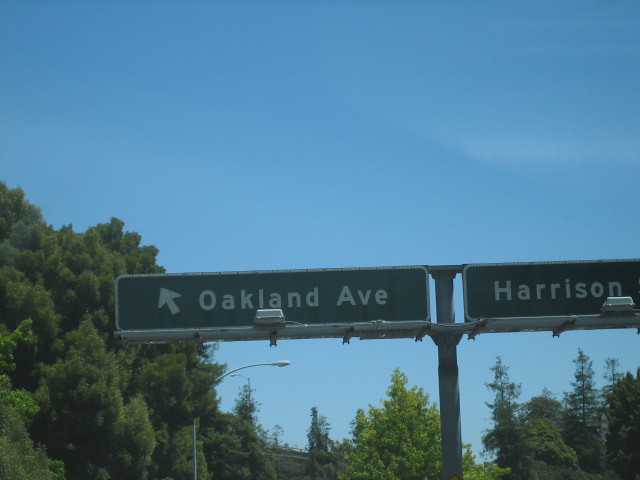The photograph captures a prominent street sign elevated high above, with the expansive sky and treetops visible in the background. The substantial pole suggests that this sign is positioned over a highway or freeway. Although the roadway itself is not visible, the context indicates a significant thoroughfare rather than a neighborhood street. The sign is equipped with lights designed to illuminate it during nighttime. In the background, there is a street lamp adding to the urban infrastructure. On the left side of the sign, "Oakland Avenue" is inscribed with an arrow pointing to the top left, possibly indicating an exit or a highway split. To the right, part of another sign is visible, reading "Harrison," but the rest is obscured. Both signs are green with white lettering, and the supporting pole is a dark grayish color.